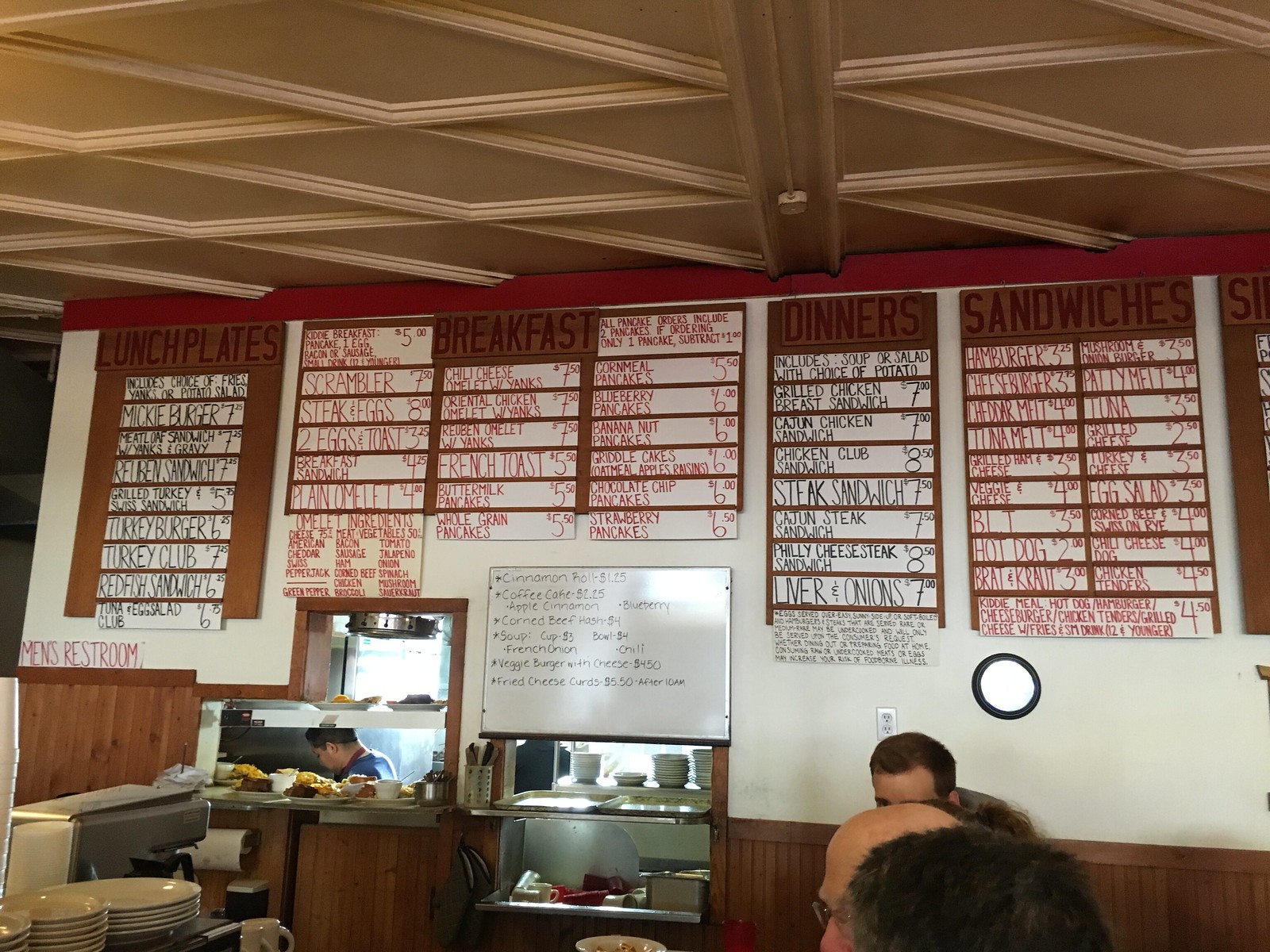This color photograph captures the cozy and inviting interior of a bustling restaurant. Dominating the upper half of the image is a series of menu boards with a charming white background framed in wood, displaying the restaurant's offerings. From left to right, the first board is dedicated to lunch plates, though the font is too small to decipher specific dishes. Adjacent to the lunch section, another panel is devoted to breakfast items, organized into three neat columns and written in red ink. Continuing to the right, a panel lists dinner options in black text, with easily readable items such as a steak sandwich and liver and onions, both priced at $7. Lastly, on the far right, there is a section for sandwiches with menu options penned in red, though the print is indistinguishable.

In the lower right corner of the photograph, the tops of three heads are visible, indicating that the restaurant is likely occupied by diners. The first head, showcasing gray hair, hints at an older individual. Beside this person, the partially bald head of a pale-skinned man is visible, alongside another man with brown hair. At the very bottom right, a glimpse of a table stacked with white dishes adds to the restaurant’s lived-in and busy atmosphere. This detailed snapshot vividly portrays the charm and variety within this eatery.